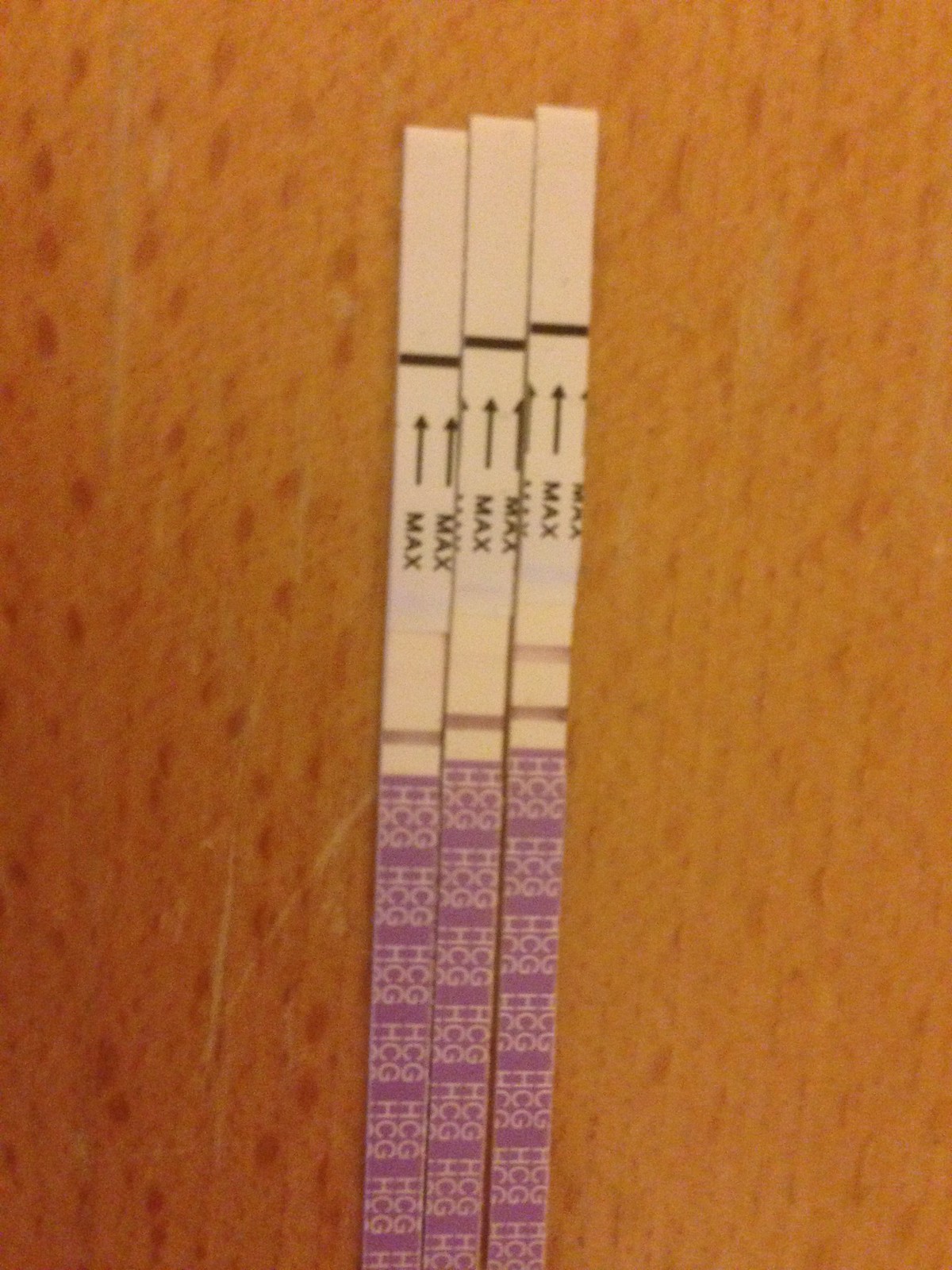This photo, taken from above, captures three identical testing strips arranged neatly in the center of an orange wood tabletop marked by light scratches. The testing strips are long and rectangular, divided into distinct sections. The upper half of each strip is off-white, while the lower half features a purple segment. Overlaid on the purple part are white letters in three sections that spell out "HCG" repeatedly.

Each testing strip also displays two occurrences of the word "MAX" accompanied by arrows pointing up toward a dark line. A clearly visible dark line is present above the word "MAX" on the leftmost test strip, indicating a result. The same layout of text, lines, and arrows is consistently repeated across all three strips. The overall image has some visual noise, giving it a slightly blurry appearance.